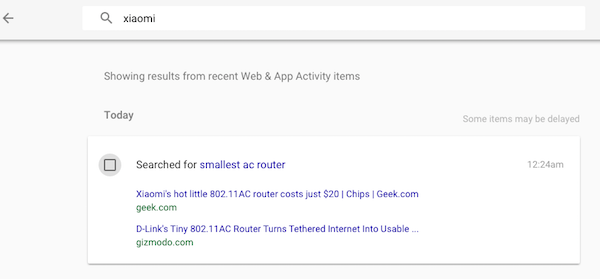**Caption:**
A detailed screenshot from a computer displaying search results for the query "Xiaomi" in an app store or internet search. At the top, a white search bar with a magnifying glass icon and the search term "Xiaomi" is prominently featured. To the left, a back icon is visible, separated by a gray line from the rest of the content below. The gray background includes text indicating "Showing results from recent web and app activity items." Below this, in slightly darker gray text, the word "Today" appears, alongside a note stating "Some items may be delayed" on the far right. 

The primary content includes a white box containing a gray checkmark next to the phrase "Searched for." In blue text, the specific searched item "smallest AC router" is shown with a timestamp of "12:24 a.m." Directly underneath, a search result snippet reads, "Xiaomi's hot little 802.11ac router costs just $20" from geek.com, along with the source in green text. Another result beneath it highlights "D-Link's tiny 802.11ac router turns tethered internet into usable..." sourced from gizmodo.com, also in green text. The overall screenshot appears to be taken from the settings displaying someone's search history.